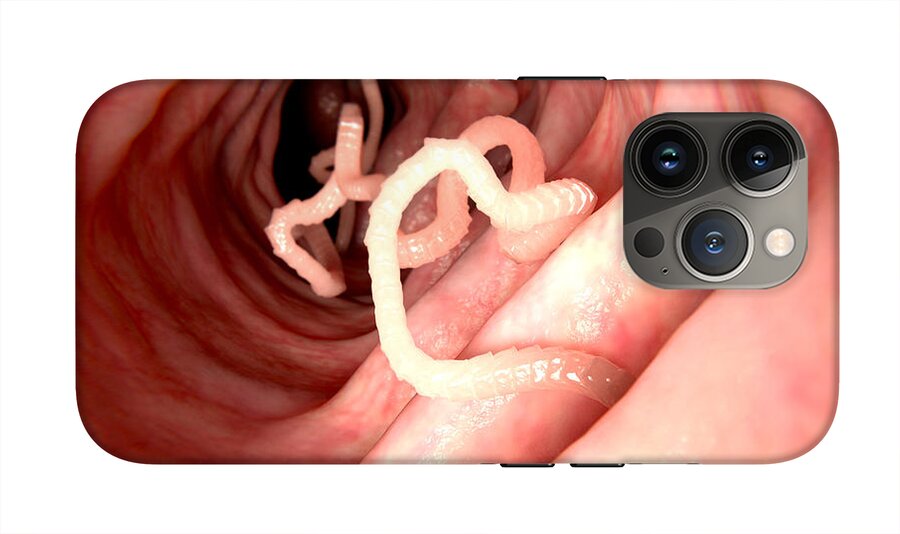The image is a detailed and somewhat unsettling mock-up advertisement for a pink, ridged phone case, featuring a unique, anatomical design. The phone is positioned horizontally with its single button facing up and double buttons facing down, placing the three-lensed camera in the upper right corner. The phone case displays a graphic that appears to be an internal view of something akin to a rectum or intestines, suggesting a medical or biological theme. The central canal of the phone case showcases numerous folds in pale creamy pink hues, transitioning to a darker brownish mauve within the folds. Winding through this canal is a worm-like entity, white and segmented, becoming pinker as it recedes into the shadows of the crevices. Additionally, the camera module on the phone, described as a black box with three circular components, adds a contrasting focal point to the intricate and bizarre design.